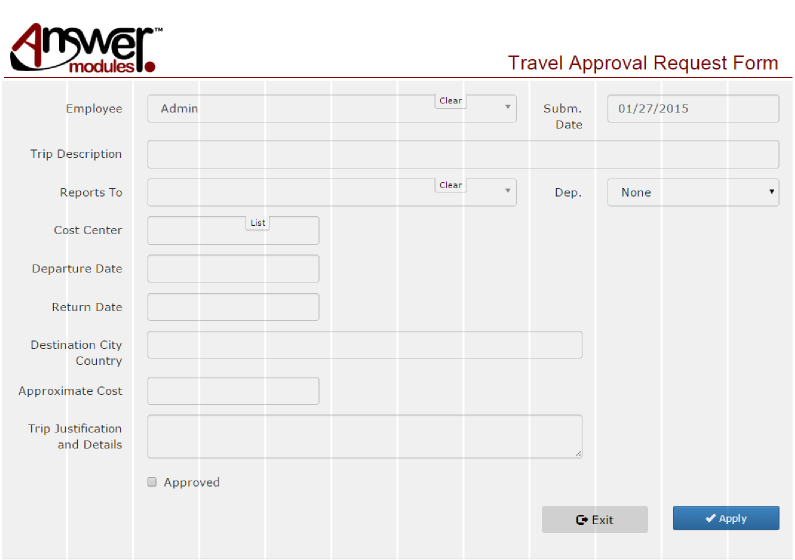This image features a horizontal web page predominantly showcasing a light gray background adorned with thin vertical white lines running from the top to the bottom. Positioned in the top left corner is the company's logo – "Answer," with "Answer Modules" written below it in black and red typeset. A thin horizontal red line underscores this logo. On the top right side of the page, the title "Travel Approval Request Form" is prominently displayed.

Aligned along the left-hand side of the image are numerous labeled boxes organized in a vertical line. These labels are presented in thin gray typeset and read: "Employee," "Trip Description," "Reports To," "Cost Center," "Departure Date," "Return Date," "Destination City/Country," "Approximate Cost," and "Trip Justification and Details." Adjacent to the "Employee" box is another box marked "SUBM Period Date," intended for the input of a specific date.

Beneath the "Trip Justification and Details" section, there is a small gray box labeled "Approved." At the lower right-hand corner of the webpage, two buttons are visible: a gray "Exit" button and a blue "Apply" button featuring a check mark.